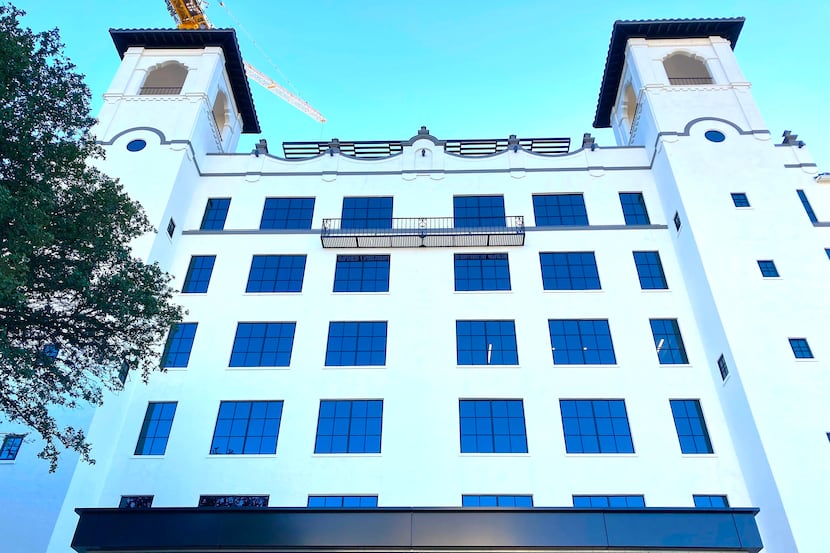This photo captures a towering, white building viewed from street level, reaching upwards against a clear, turquoise sky. The image does not include the ground, emphasizing the structure's impressive height and the two prominent square-topped towers on either side. Each tower is topped with navy blue, protruding roofs and features large, open windows framed by black railings. Between the towers, the main building facade is lined with five stories of large, square blue glass windows framed in black, arranged in a grid pattern. Alongside these are slim, vertically rectangular windows. There is a visible black overhang at the bottom of the image and a black scaffolding structure, likely for window maintenance, attached around the fourth or fifth level. To the left, a tree with green leaves partially intrudes into the frame. At the top left corner, a yellow crane is positioned as if engaged in ongoing construction work.